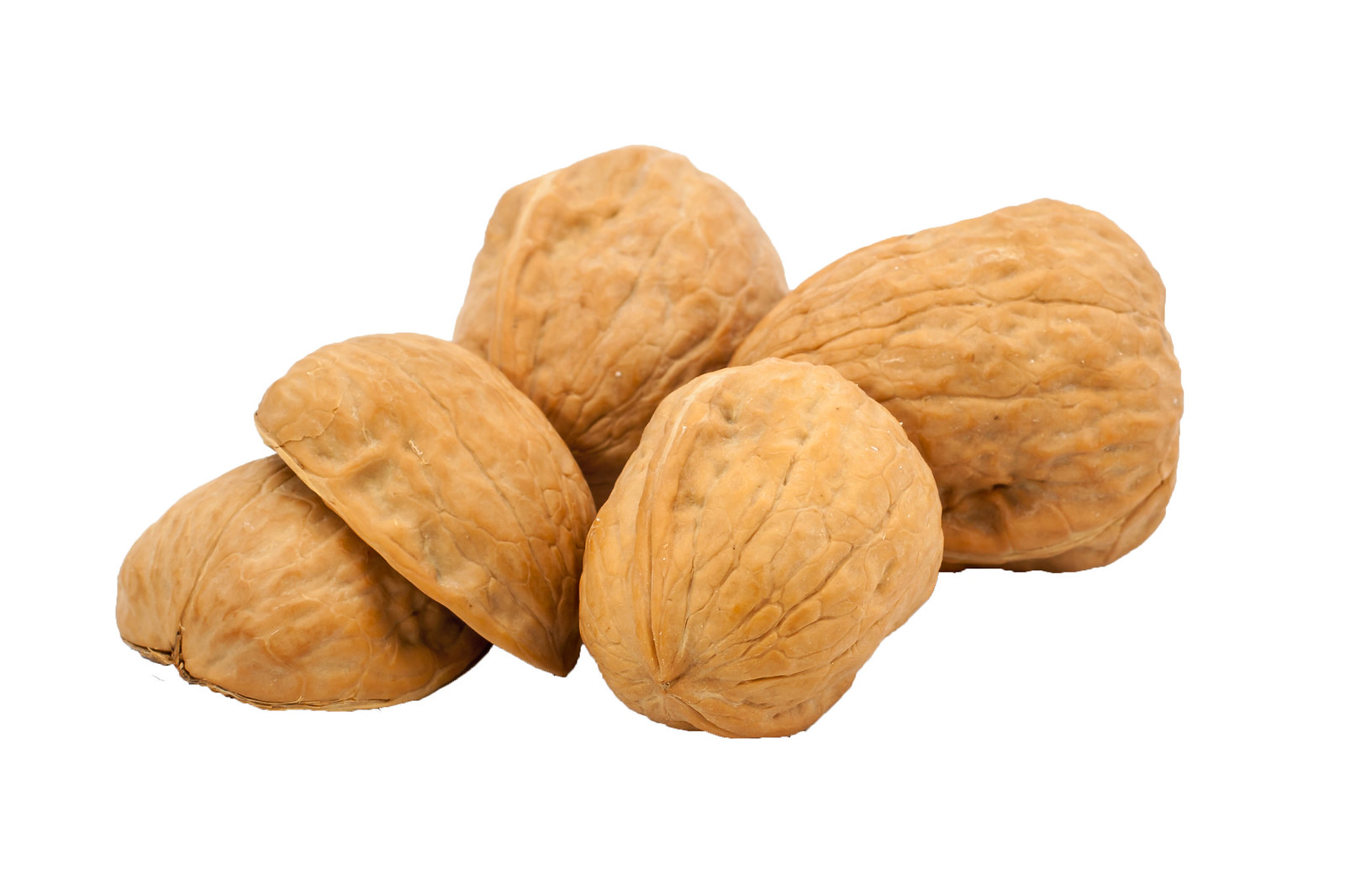This high-resolution, close-up photograph showcases four walnuts in their shells against a stark white background. The image is well-lit, emphasizing the light brown, tan, almost sandy beige color of the walnut shells. The walnuts have an oblong shape, slightly larger at one end, and feature a characteristic fissure around their circumference, which aids in cracking them open. Three whole walnuts are arranged in the image—two in the back and one in the foreground, with one facing the camera directly. The fourth walnut shell is split into two halves; one half lies flat while the other is perched jauntily atop it like a cap. The meticulous arrangement and sharp focus suggest a product image suitable for a website, highlighting the texture and natural design of the walnuts.